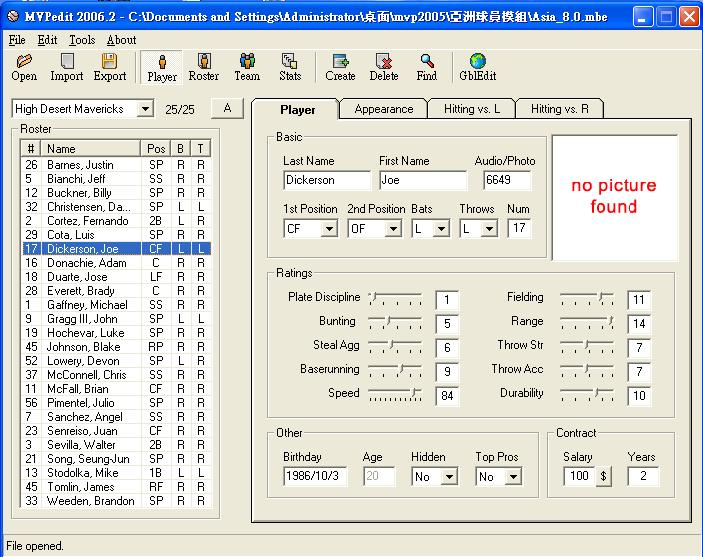The image is a detailed screenshot of an old sports management software, MVP Edit 2006, running on a Windows operating system. The program window, reminiscent of classic Windows with its blue title bar and red 'X' close button, displays the path "C:\Documents and Settings\Administrator\[...] (Chinese text)\MVP 2005\[more Chinese text]\Asia_8.0.MBE" at the top. In the top left corner, there's an icon of a baseball, indicating the application's focus on baseball management.

The main interface features several menus and buttons labeled File, Edit, Tools, and About, along with options like Open, Import, Export, Player, Roster, Team, Stats, Create, Delete, Find, and Global Edit. The left pane lists various players from a team named "Hi Desert Mavericks," with the name 'Joe Dickerson' highlighted, showing his position as CFLL (likely center fielder, left-left handed).

The right pane provides comprehensive details about Joe Dickerson, including editable fields for his name, photo (currently showing "no picture found"), stats like plate discipline, bunting, steal, average, base running, speed, fielding range, throwing stats, birth date (October 3, 1986), age, and contract information ($100,000 salary for two years). Additionally, there are specialized stats labels such as hitting versus L (left) and hitting versus R (right). This thorough database interface suggests the software is used for detailed player management, possibly for setting up game rosters or analyzing player performance.